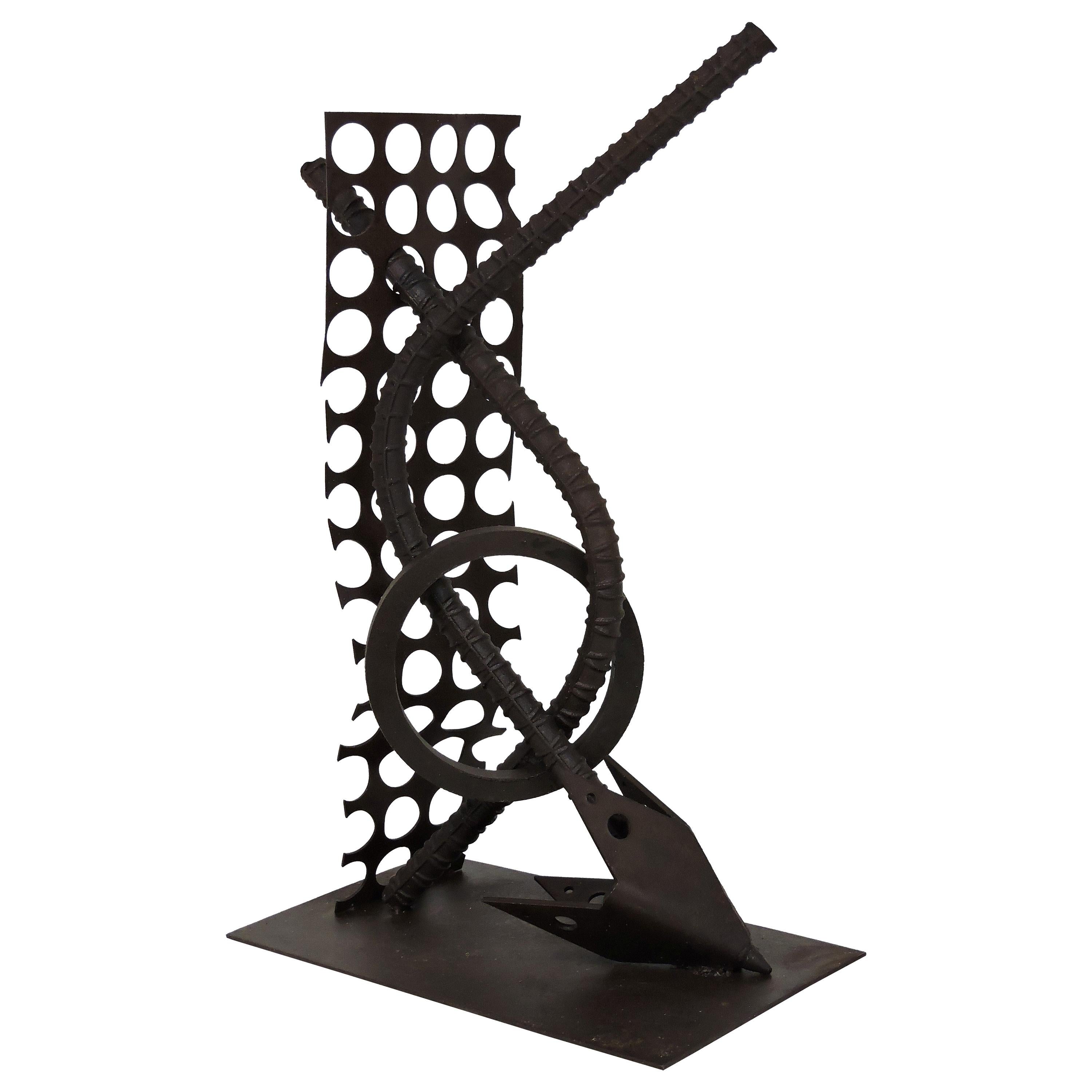This photograph features a striking modern metal sculpture set against a stark white background. The sculpture is primarily black and composed of several meticulously shaped and welded elements. The base is a thin, rectangular black plate that provides support for the structure. Attached to the left side of the base is a taller, more slender rectangular piece, also black, riddled with an orderly array of holes in a 4 by 12 pattern.

Central to the artwork is a large diameter rebar, bent and painted black, that spirals and curves intricately around the sculpture. This rebar forms loops and passes through a prominent ring. Where the rebars intersect, one extends into a pointed end, reminiscent of an arrow or spear, evoking imagery of weaponry or possibly rocket fins.

The rebar configurations include a secondary piece that coils within the loop of the primary rebar, adding to the layers of complexity. This entire composition creates a sense of movement and interaction between the various metal elements. Despite its industrial materials, the sculpture conveys a sense of fluidity and dynamic energy, emblematic of contemporary artistic interpretations.

The overall impression is one of an elaborate, thoughtful piece of modern art that draws the eye to its coiling forms and intersecting lines, all highlighted beautifully against the clean, white backdrop that serves to emphasize its intricate, black-painted details.